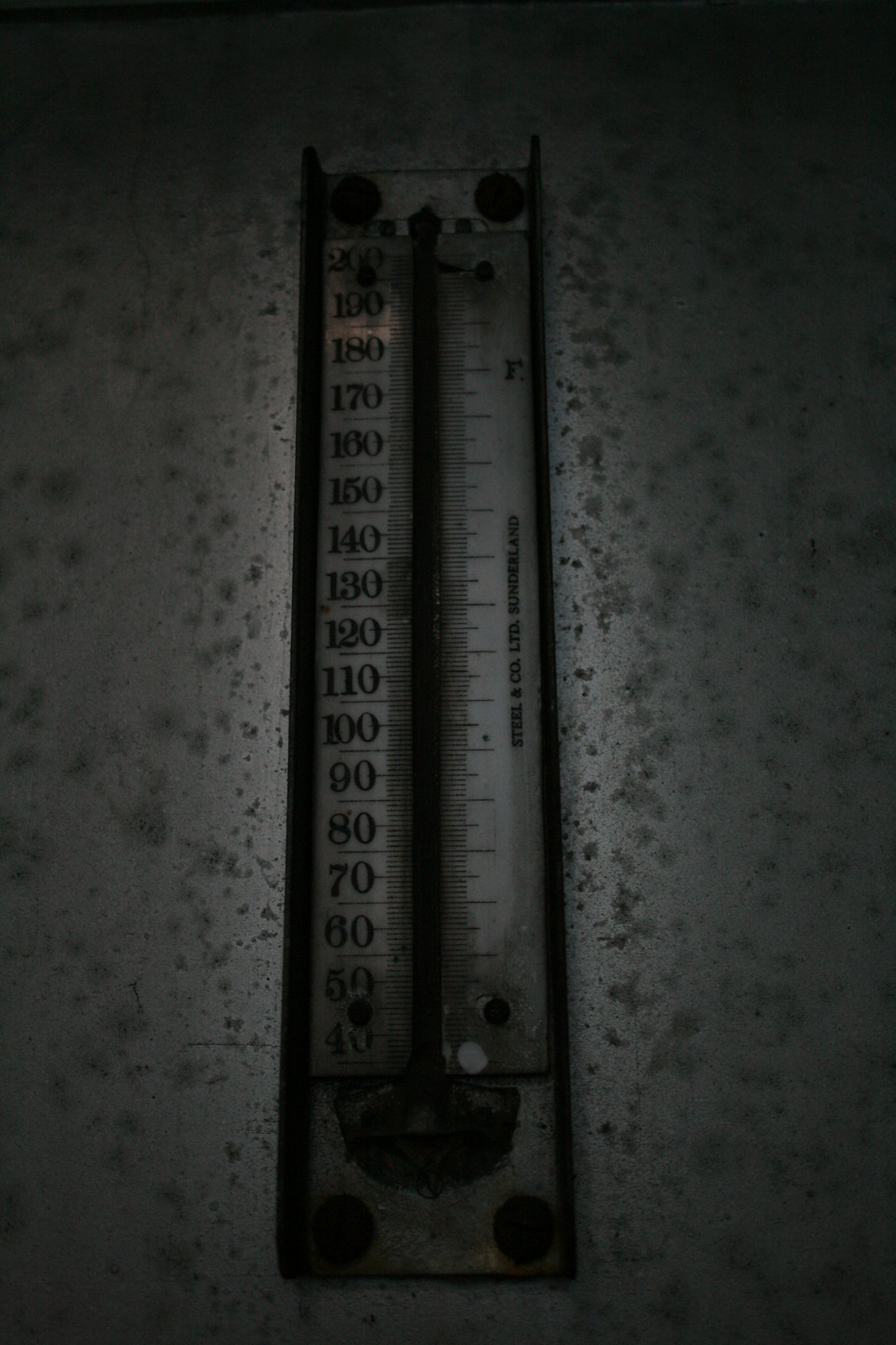The image is dark and features a central object that appears to be an old thermometer or gauge. The backdrop is a white surface, speckled with gray dots of varying shapes. Shadows heavily dominate the top, sides, and center of the image, contributing to the overall dark appearance. 

The central object—a long, possibly antiquated thermometer or gauge—displays numerical markings, starting from 200 at the top and decreasing by tens: 190, 180, 170, and so forth, down to 50. Below the 50 mark, the image is too dark and shadowy to discern any further details. The gauge itself is long and black, with no other distinguishable colors.

On the right side of the gauge, the white background features several lines running vertically, some long and some short. Near the far right side of the gauge, there is a bit of black text, although it is not clear enough to read. The contrasting shadows and speckled dots on the white surface, along with the detailed numerical markings and lines, create a complex and visually intriguing scene.